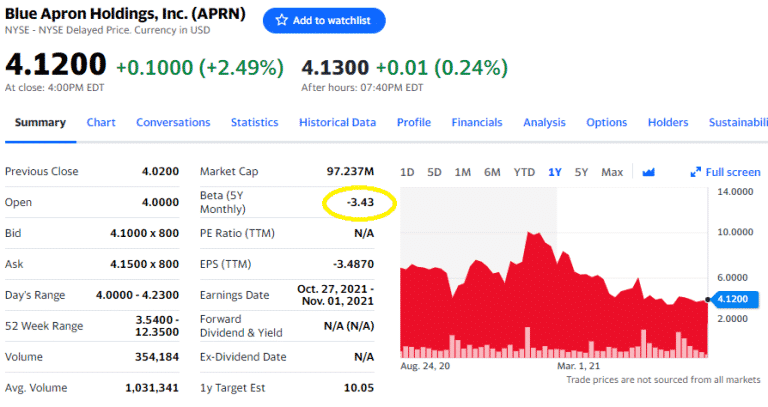This is an image of a stock page with a predominantly white background and black headers. At the top, it reads "Blue Apron Holdings Incorporated (APR)." To the right of this, there is a blue tab labeled "Add to Watch List" accompanied by a star icon. Beneath the company name, the text "NYSC - NYSC Delayed Price. Currency in USD" is noted in black font.

Directly below this, the current stock price is displayed as "4.1200" in black, followed by a green figure "+0.1000" and "+2.49%" in parentheses, indicating the percentage increase. Towards the bottom right of the image, the stock chart is displayed in red, depicting fluctuating data. Above the chart, various time frame options are listed: "1 Day, 5 Day, 1 Month, 6 Month, YTD, 1 Year, 5 Year, Max," with the "1 Year" option highlighted in blue.

To the left of the chart, additional stock details are provided, such as "Previous Close, Open, Bid, Ask, Day's Range," along with their respective values. Positioned above these details and beneath the stock price of "4.1200," there are tabs for further information: "Summary, Chart, Conversations, Statistics, Historical Data, Profile, Financials, Analysis, Options, Holders, Sustainability."